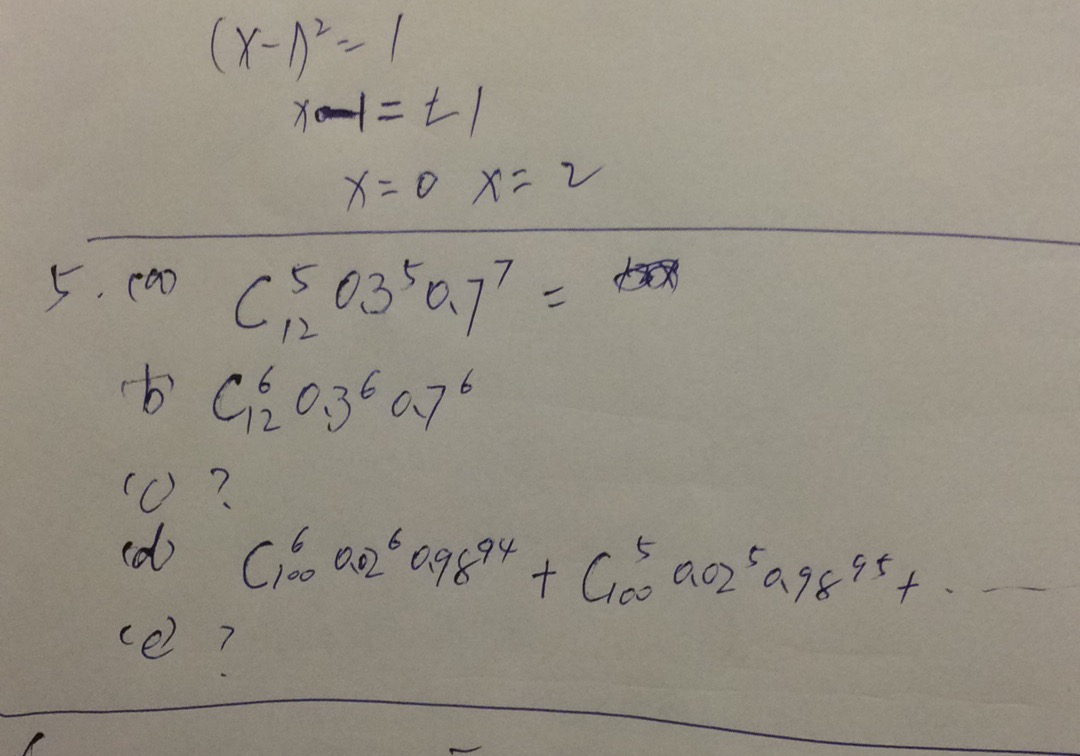This image captures a sheet filled with complex calculations, written on what appears to be a piece of white paper, though it has a slight lilac-gray tint in the photograph. At the top, there's an equation: \((x-1)^2 = 1\), which leads to solving \(x-1 = \pm1\), giving the solutions \(x = 0\) and \(x = 2\). A prominent horizontal line separates this section from the rest of the notations below.

Further down, there are numerical expressions and calculations meticulously noted. There's a sequence starting with \(5.00C_{5}^{12}0^3 \cdot 7^7\), followed by a scribbled-out section. Below this, another term: \(\frac{(T O C)^6}{12} \cdot 0.36 \cdot 0.7^6\), is inscribed. The notation continues on subsequent lines with mixed letters and numbers, incorporating parentheses and question marks that suggest uncertainties or placeholders in the computation.

There is also a specific segment marked with \( (D) \frac{C6}{100} \cdot \frac{0}{02^6} \cdot 0.98^{94} + C_{100}^5 \cdot 0.02^5 \cdot 0.98^{95} + \ldots \), illustrating a complex series sum or probability calculation. This part is followed by another line indicating \( CE^7 \), ending with a question mark, and is concluded by another long line across the page, perhaps signifying the end of the calculations or a section break. These intricate notations and symbols suggest an advanced mathematical or statistical analysis, filled with variables, exponents, and constants.